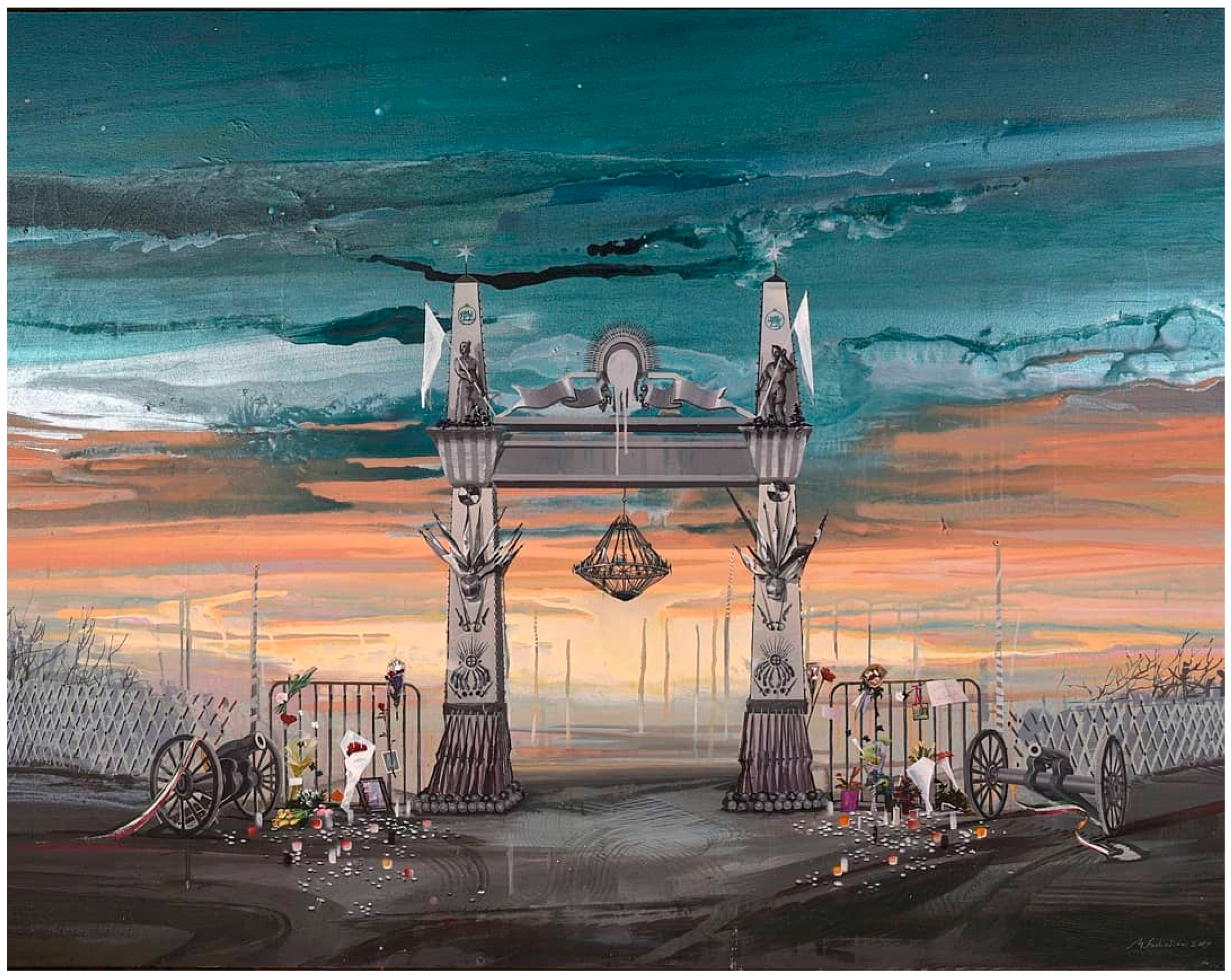The artwork, a striking watercolor painting, portrays a grand and detailed entrance gate set against a dramatic, ombre sky transitioning from a turquoise blue to a deep orange, suggestive of a sunset. The sky, pronounced by detailed clouds, fades into an orange hue, creating an ethereal atmosphere. The gate, the focal point of the composition, consists of tall, sturdy columns connected by an arch-like horizontal beam. Suspended from the center of the beam is a chandelier or dreamcatcher-like object. Each side of the gate is adorned with potted feathers and flowers, hinting at a ceremonial or memorial significance. Below, the barren and grey terrain contrasts sharply with the vibrant sky, and two battlefield cannons stand guard beside each column. Statues resembling Native American figures holding white flags are positioned on the beam, signifying peace or tribute. This intricate gateway, possibly symbolizing a passage to another life or realm, evokes a mysterious and poignant scene, rich with cultural motifs and historical elements.